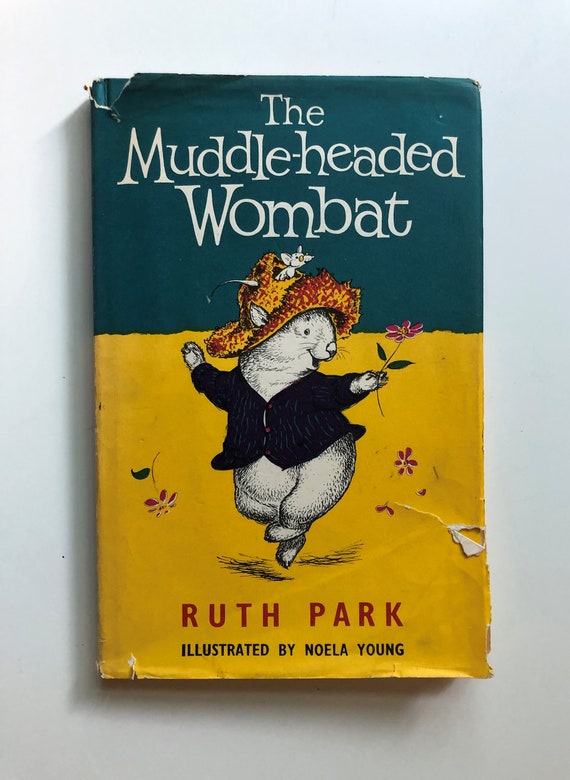The image is a photograph of an old book cover, set against a white background that might be a table. The book is titled "The Muddle-Headed Wombat" by Ruth Park, illustrated by Noella Young. The paper cover is noticeably worn, with tears revealing a dark teal underlayer in the top left corner. The title is in white text on a dark teal background that stretches from the top left to the top right. The author's name, Ruth Park, is written in red text towards the bottom, alongside the title in black text on a mustard-yellow background.

The central illustration features a cheerful, furry wombat, likely from Australia, standing upright and looking towards the right. The wombat is depicted in a jubilant pose, appearing to jump or skip in the air. It is dressed in a black jacket and an orange hat with holes through which its ears poke out. A small mouse, wearing glasses, peeks out from a hole in the hat, adding a charming touch. The wombat holds a pink flower with green leaves in its right hand. The illustration is complemented by a floral background, also featuring a mustard-yellow hue, with some flowers seemingly falling off the character.